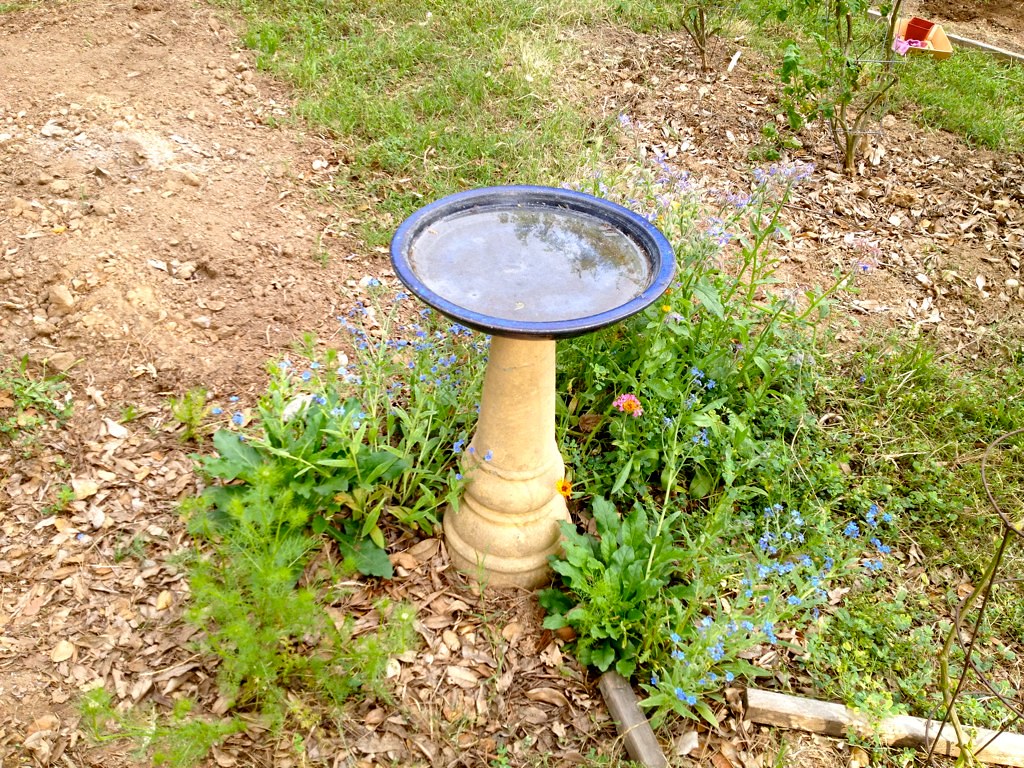This photograph captures a birdbath in an outdoor garden-like area. The birdbath features a yellow concrete-looking base that tapers at the top and widens at the bottom for stability. Atop the base sits a purplish-black saucer filled with water, positioned directly on the bare ground. Surrounding the birdbath is a mix of dirt and flowering weeds, including very small pink and purple blossoms. In the upper right corner of the image, a small tree or two can be seen growing out of the dirt. Additionally, the background reveals a yellow and red object, possibly a child's toy or some lawn decor, situated on a patch of grass.